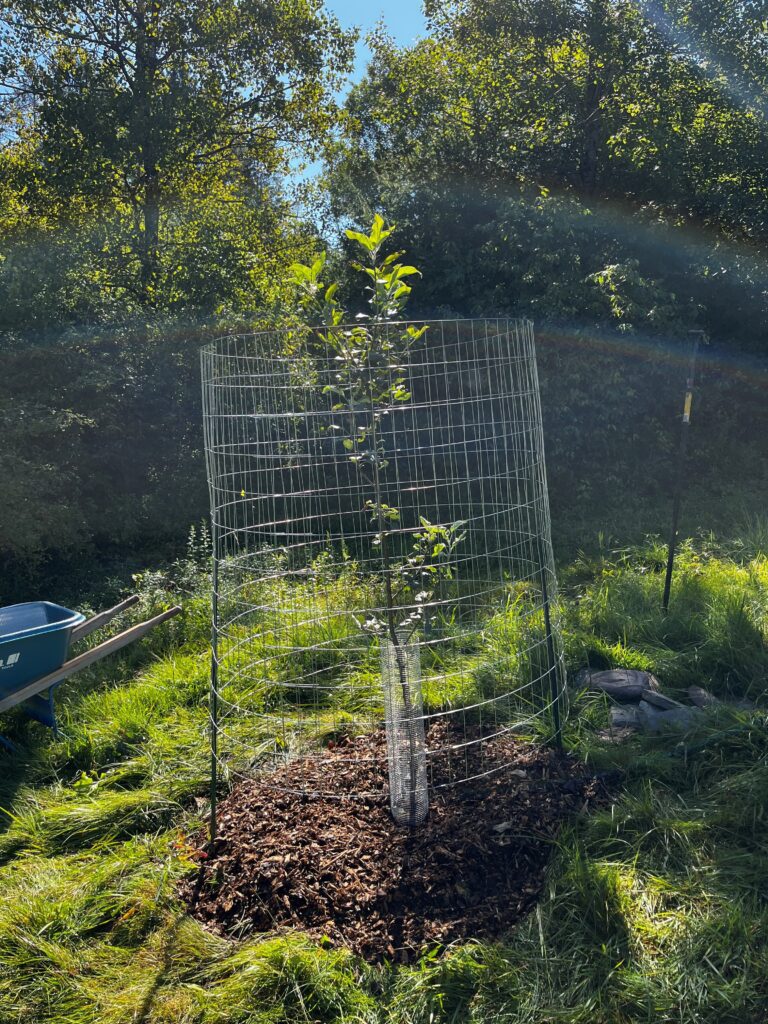In this outdoor image, set possibly in a backyard or front yard, the focus is on a small plant centrally planted in the ground. The base of the plant is encased in some kind of plastic wrap, which is secured into the soil. The plant is tender, with green leaves sprouting from the top, and is protected by a cylindrical silver-like fence encircling it. Surrounding the base area is a patch of fresh soil, emphasizing its newly planted status. To the right of this soil patch is a cluster of gray stones, offering a contrast to the earth tones of the scene. On the left side rests a small blue wheelbarrow with wooden handles jutting out, adding a touch of rustic charm. The background is lush with green trees and bushes, framing this serene garden setting with natural vibrancy.